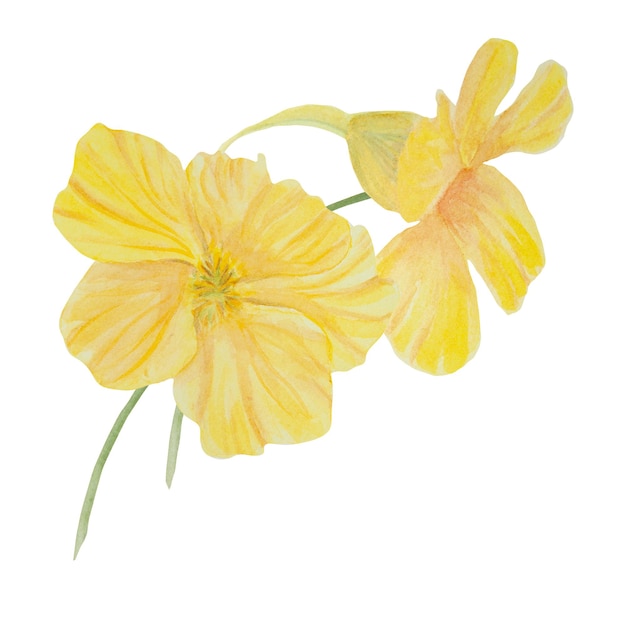The image depicts a delicate watercolor painting of two yellow flowers set against a plain white background. Both flowers have thin green stems. One flower is directly facing the viewer, showcasing five or six large, striated petals that are predominantly yellow with subtle shades of pink, adding depth and texture. The second flower is oriented to the viewer's right, revealing the back of the bloom with more pronounced pink hues towards the center. This flower also features a rear petal extending outward. The artist used layers of white, faint yellow, and a darker mustard yellow for petal striations and shadows, along with hints of peach to soften the overall tone. Although the exact type of flower is unidentified, it has a common, garden-fresh appearance similar to those seen annually in Minnesota gardens.